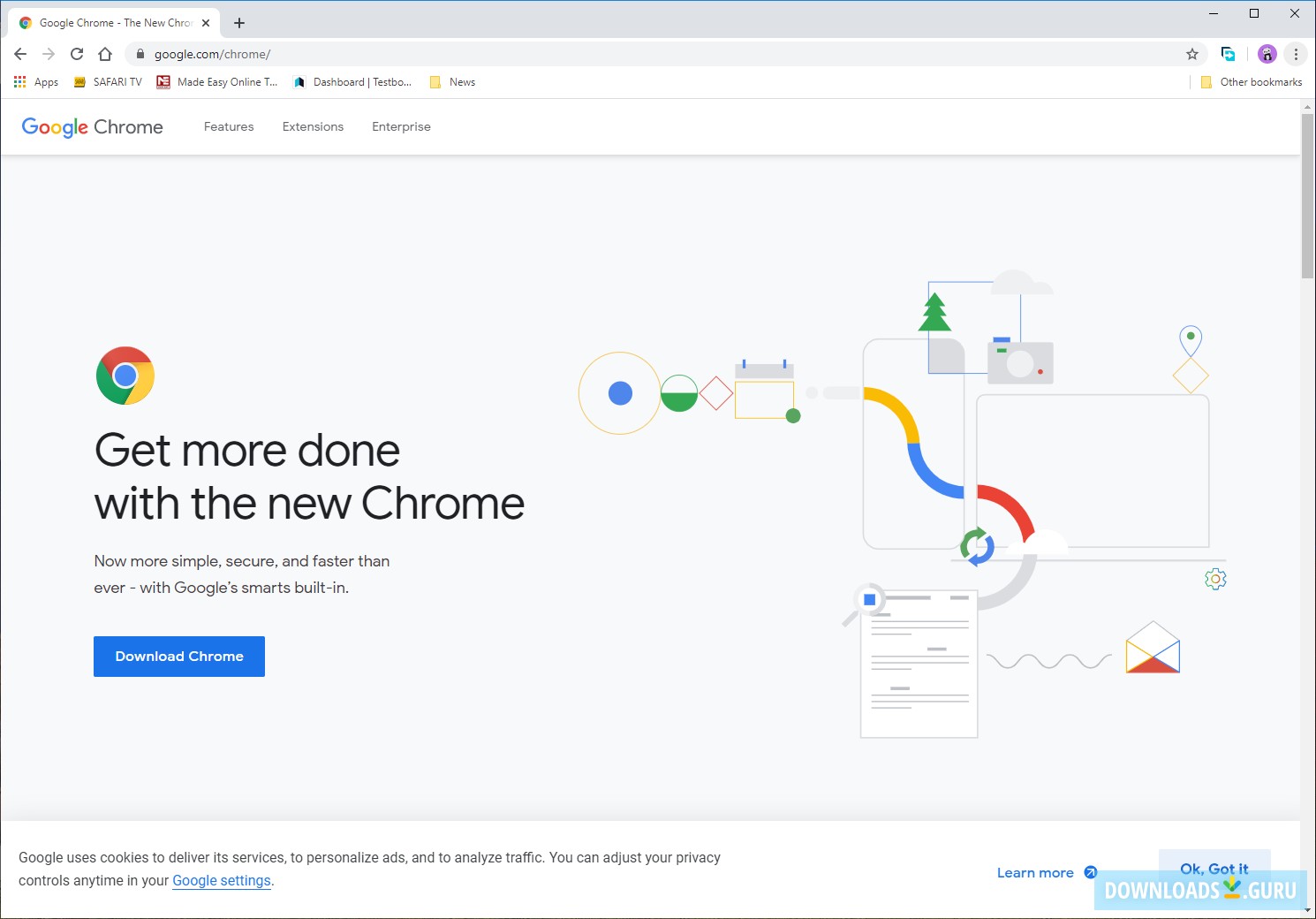### Detailed Caption:

The image illustrates a promotional graphic for the new Google Chrome browser, inviting users to enhance productivity. Central to the design is the iconic Google Chrome logo—a circle segmented into red, green, and yellow sections, with a blue dot in the middle. Adjacent to this emblem, three colored lines (yellow, blue, and red) meander through two squares, adding a dynamic visual element.

Above this, a green pine tree is featured, symbolizing freshness or new growth. Additionally, a grey camera with a blue button and a red light is depicted, possibly suggesting multimedia capabilities. Below, a uniquely designed red envelope consists of a red base, a red triangle, two inward-pointing white triangles, and a white diamond at the top, indicating messaging or email functionalities.

At the bottom of the image, there is a disclaimer stating, "Google uses cookies to deliver its services, to personalize ads, and to analyze traffic. You can adjust your privacy controls anytime in your Google settings," with "Google settings" highlighted in blue. There is also a "Learn more" link.

In the lower right corner, the text "Downloads Guru" and an “Okay, got it” button are present. The image displays a URL at the top left and an “X”, maximize, and minimize buttons at the top right. Additional icons and text suggest various browser features, extensions, and enterprise options, including bookmarks, news, online tools, Safari TV apps, and buttons for refreshing, navigating backward, and forward.